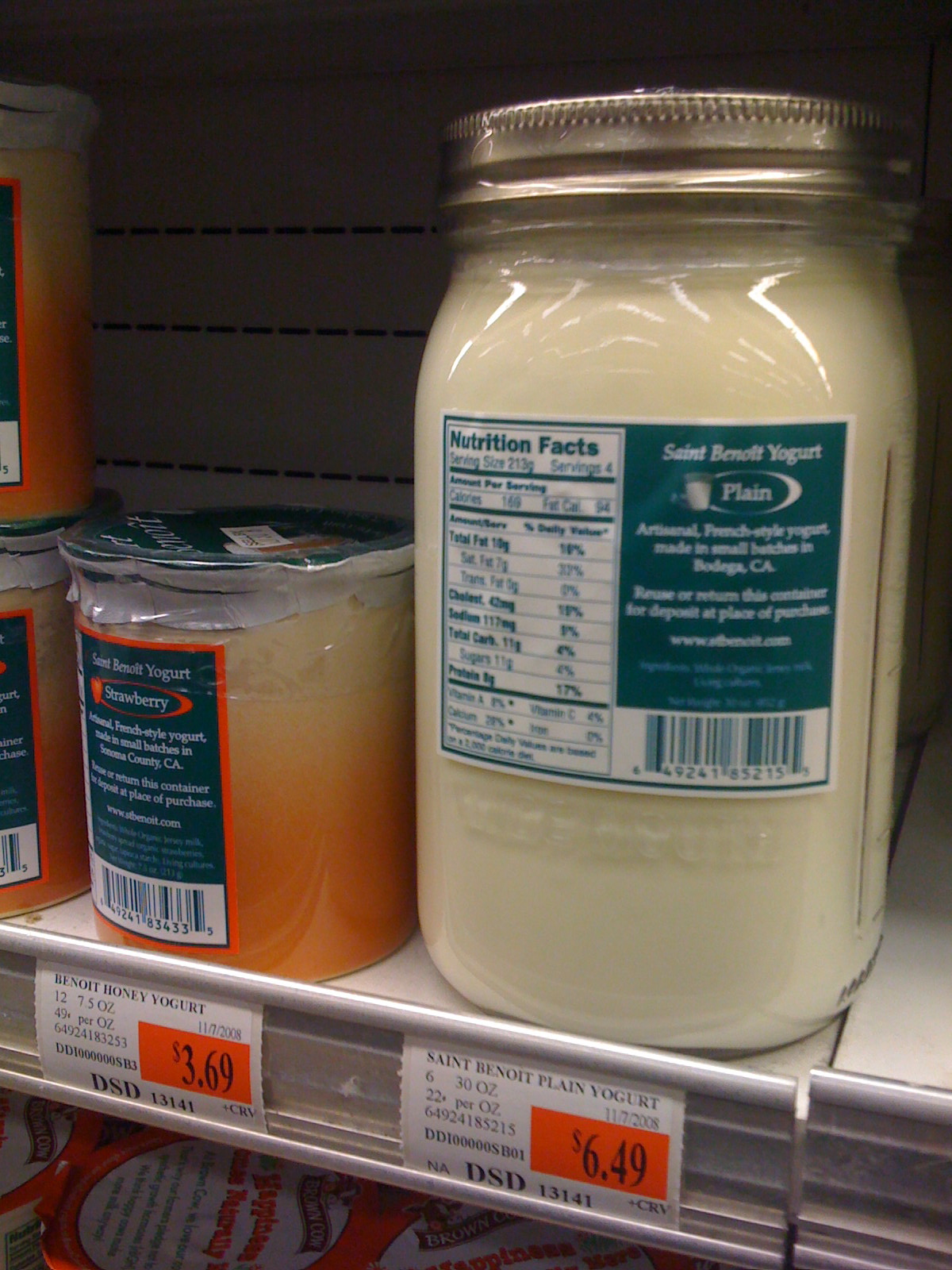This is a color photograph taken indoors in portrait mode, depicting a grocery store shelf with a metal rim for holding price tags. On the shelf are two jars of St. Benoist yogurt, each with a distinct appearance and label. The jar on the right is a tall, clear glass jar containing a whitish creamy substance and has a brass-colored metal screw-top lid. The front-facing label indicates "Saint Bruno Plain Yogurt" priced at $6.49, with additional details such as it being made in California, and displaying nutrition facts. The jar on the left is a shorter, clear glass container with an orange substance at the bottom and plain yogurt on top, suggesting it needs to be stirred. It is sealed with a green plastic lid and labeled "Saint Bruno Yogurt Strawberry," priced at $3.69. The background consists of a slat wooden wall, and partially visible products are stacked next to and below these jars.